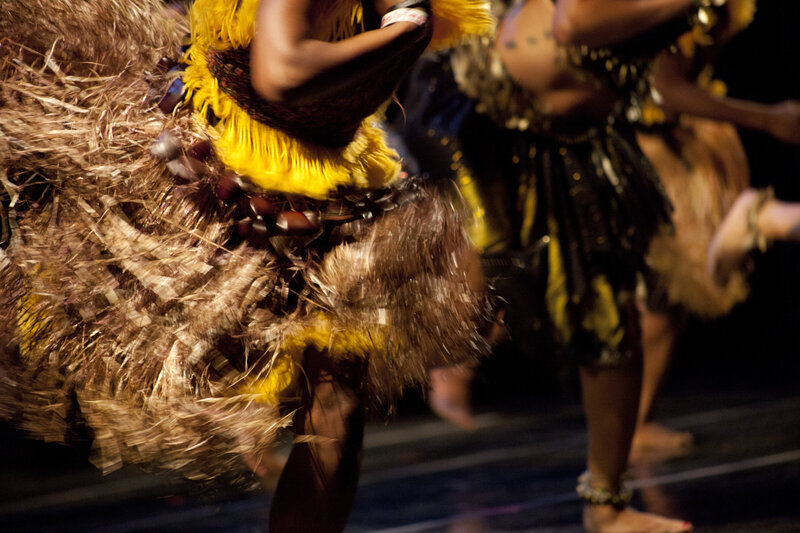This close-up photograph captures a dynamic scene of island dancers adorned in traditional Pacific Island or Polynesian attire. The image primarily focuses on their movement, showing three dancers from the shoulders down, all seemingly caught in mid-motion as they dance on a black floor against a dark backdrop. Their bare feet suggest an energetic dance, possibly a shuffle, jump, or similar movement.

The dancers' costumes are intricately detailed, made primarily of straw-like or woven plant materials in shades of yellow and tan, reminiscent of taxi cab colors. The outfits feature yellow strings or ribbons and are accessorized with belts of large wooden beads and strings of shells around the ankles. One male dancer is shirtless, wearing only a vest-like garment around his chest, while another has a vest with yellow string accents. The yellow and brown hues of their attire highlight the traditional and cultural essence of the dress. The dancers' skin tones range from light brown to dark, enhancing the rich diversity and cultural authenticity depicted in the photograph.